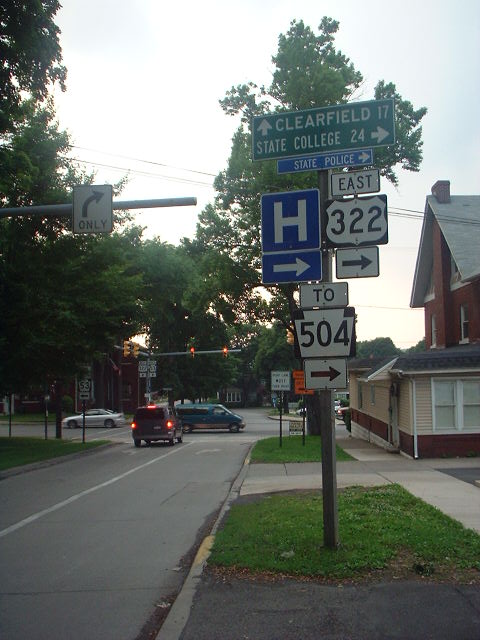A suburban intersection bustling with activity is captured in this detailed photograph. Three cars are visible, navigating the crossroads, surrounded by an array of street signs providing directions and information. Prominent among the signs are green directional boards indicating distances: Clearfield is 17 miles away, while State College is 24 miles. An additional green sign directs travelers to the State Police on the right. The intersection is marked by a highway sign for East 322, alongside symbols for a hospital (H) and route marker 2504, all pointing to the right. Above the right lane, a sign clearly mandates a right turn only, a directive also painted on the road surface. To the right of the intersection, a house, a well-maintained sidewalk, and a patch of grass lend a suburban character to the scene, distinguishing it from a typical highway environment.